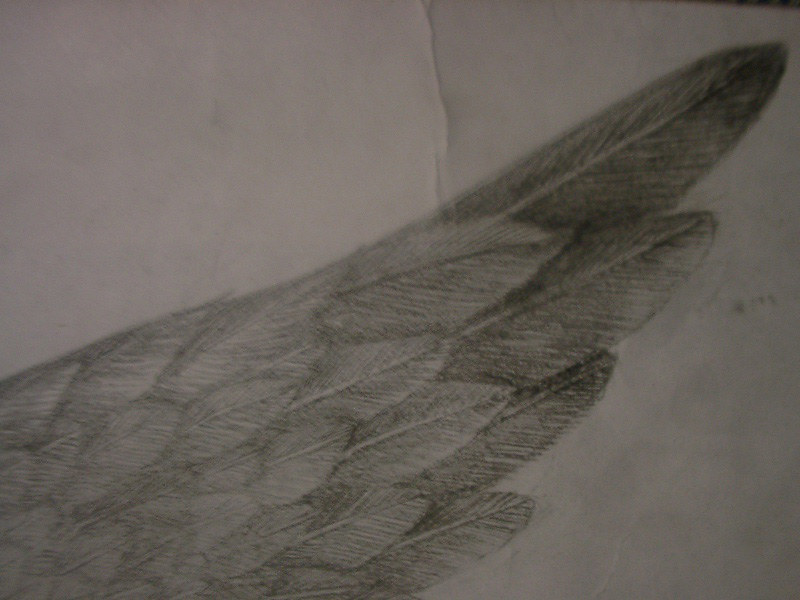This image features an extremely zoomed-in sketch, either of a bird's wing or a cluster of leaves. Starting from the bottom left-hand corner, a series of leaf-like shapes are meticulously shaded in gray. These shapes are smaller at the beginning and gradually increase in size toward the right. The last few shapes are notably darker and larger than the rest. The background consists of gray paper, with a prominent creased line running vertically down the center from the top. In the top right corner, there is a subtle hint of a black background, adding depth to the overall composition.